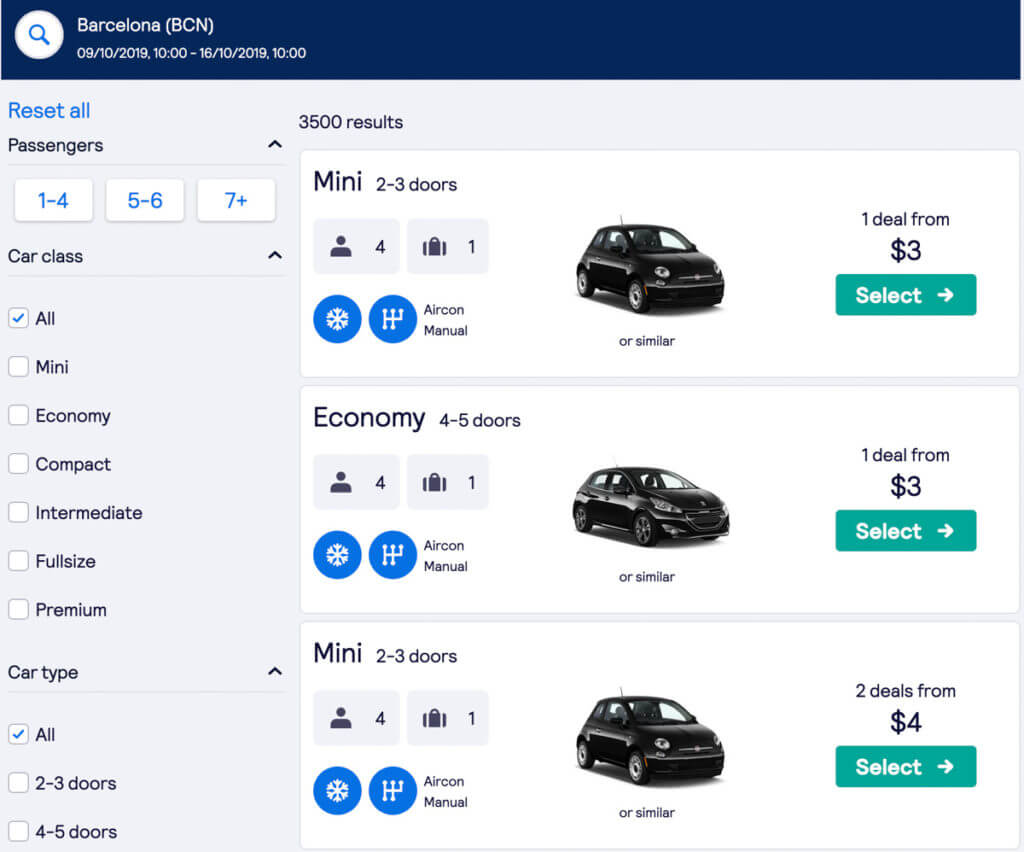Captured in Barcelona on September 10, 2019, at 10:00 AM, this image features an intricate arrangement of curly strings. The setting and photographic details suggest a busy time and place, possibly near a transportation hub given the mixed details about car classes and rental deals. The description also oddly includes a variety of rental car options such as mini, economy, compact, intermediate, full size, and premium, with specifics mentioning deals for mini (starting at $4) and economy cars (starting at $3). This detailed mishmash hints at a juxtaposition of abstract elements against the structured backdrop of transportation logistics.